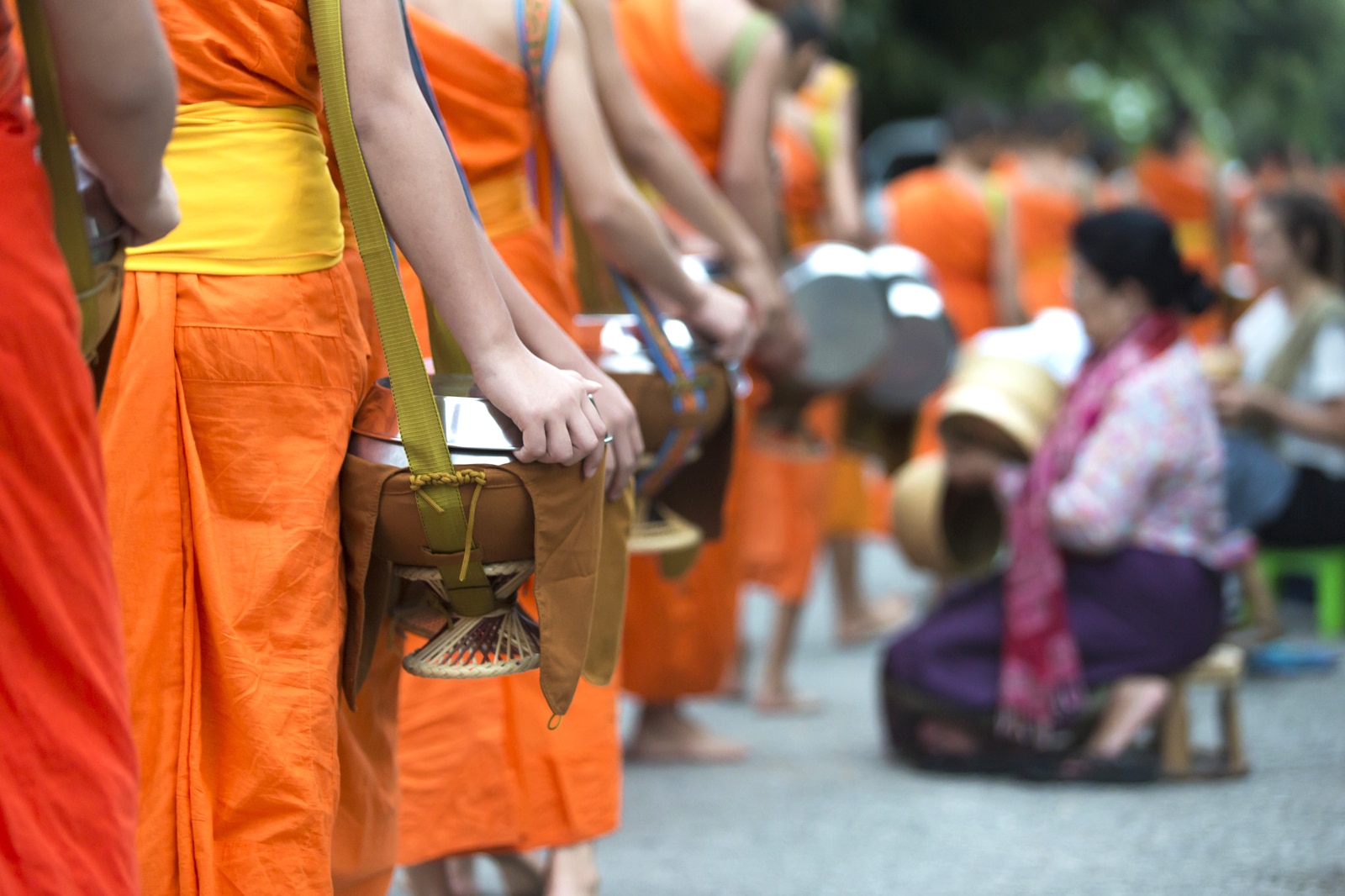The photograph captures a fairly large group of women, possibly monks, standing in a curved line. They are adorned in vibrant orange robes, with some wearing shades of red, and have gold sashes or belts tied around their waists. Draped over their right shoulders, they carry what appear to be drums with a brown base and a silver metal top, resembling urns or pans on straps. The image is mostly taken from behind, showcasing their right arms and shoulders. The background is blurry but features an elderly woman in a dark purple skirt, a pink top, and a dark pink scarf, kneeling on a small stool while holding a golden container or basket. Further off in the distance, more women in similar orange attire can be seen. The setting appears to be outdoors on gray asphalt, surrounded by trees, suggesting a ceremonial or ritualistic gathering, possibly of Indian or Asian origin.